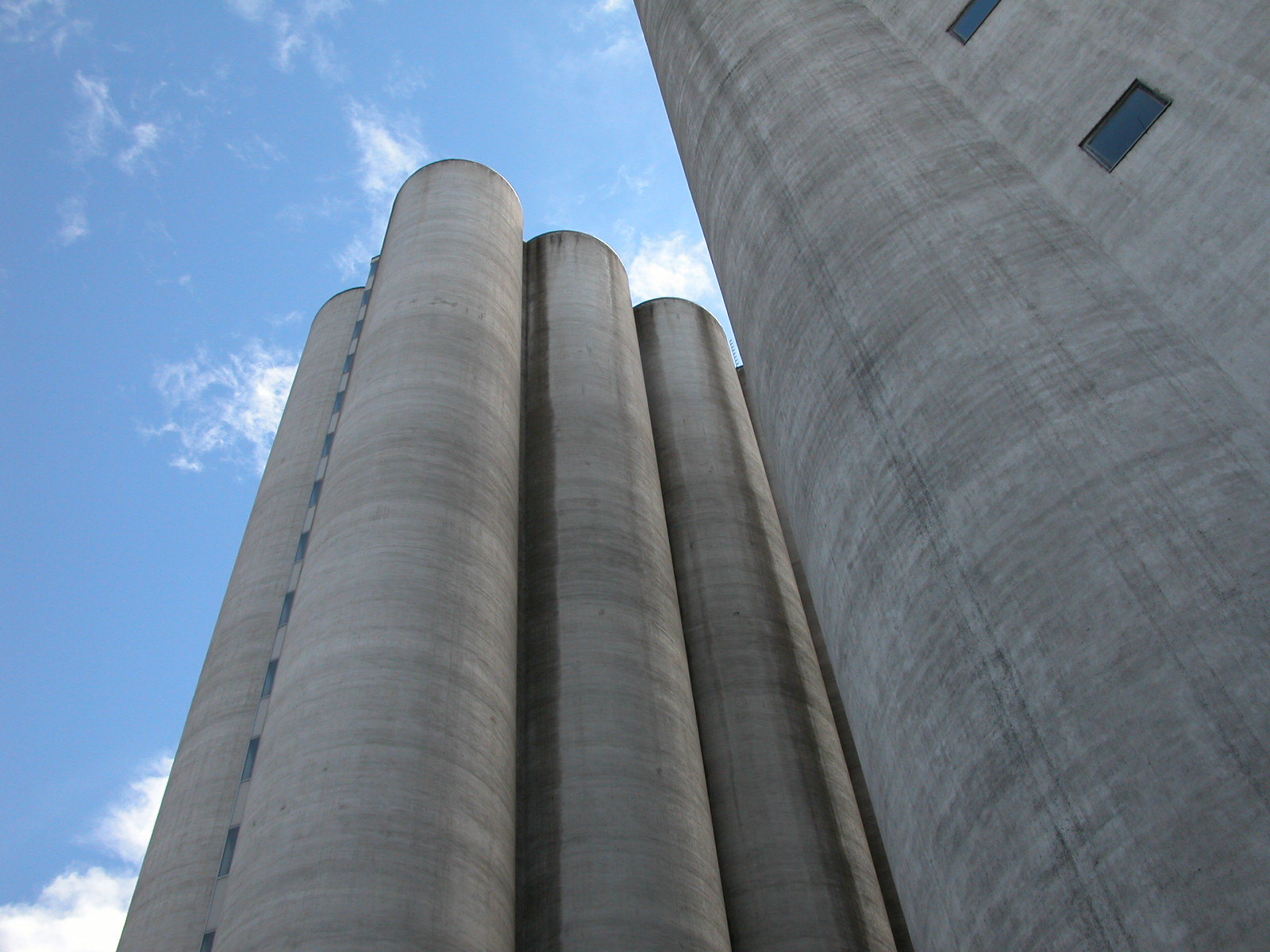This photograph, taken outdoors on a clear day with a bright blue sky dotted with fluffy white clouds, captures the perspective of looking up from the ground. The image centers on a factory-like structure composed of several very tall, cylindrical, gray cement columns. These tubular columns are grouped closely together, resembling storage containers, pipes, or possibly smokestacks, commonly seen in industrial settings such as factories or refineries. The structure, devoid of text, features a few small square windows on the left and possibly rectangular windows on the right, although these could also be design elements. The imposing gray cylinders stretch high up into the sky, emphasizing the monumental scale of the industrial architecture.